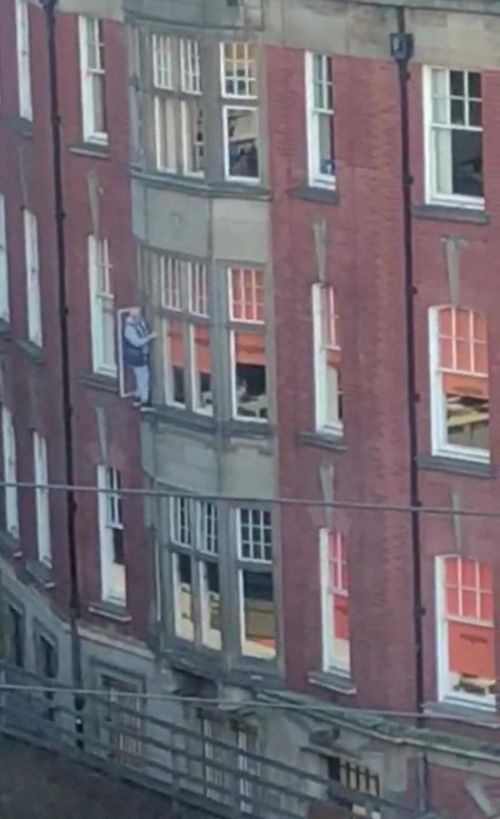The image depicts the exterior of a several-story, red brick building. The view shows at least three floors visible, along with potential glimpses of a basement level. A cathedral-style window is prominently featured, where on the ledge of what appears to be the third floor, a man is precariously positioned. This man, who looks older and is wearing a blue jacket with gray sleeves, jeans, and black shoes with white soles, is standing with his backside to the open area. He is holding onto the window frame with his right hand while looking over his right shoulder, giving the impression he might jump. The windows of the upper floors are lit from within and display a variety of interior colors, including pink, white, and tan. Below this scene, a couple of power lines and a railing are visible, further adding to the urban setting of the image.